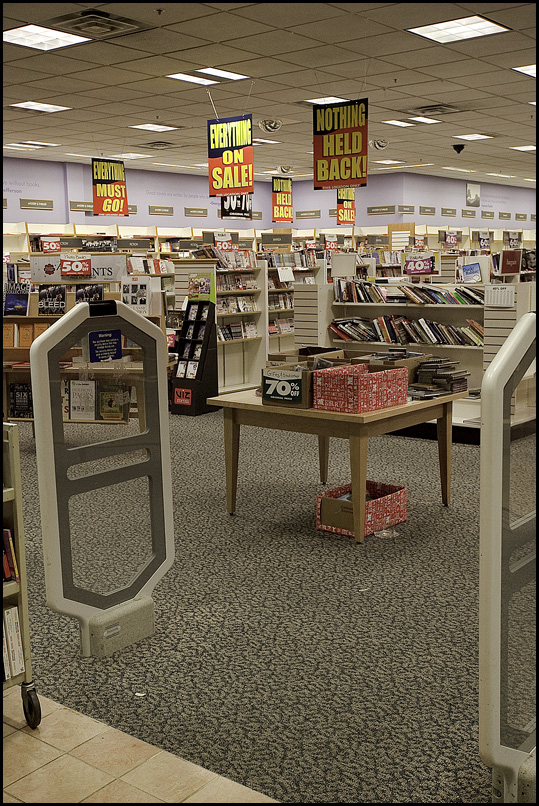The image depicts the interior of a large bookstore that is in the process of closing down. From the forefront, we gaze past the security scanners typically used to deter theft. We stand on a tiled entryway that transitions into a carpeted floor throughout the store. The bookstore is filled with numerous shelves, many of which are somewhat disorganized with books haphazardly stacked. Prominent signage hanging from the ceiling proclaims, "Everything must go," "Everything on sale," and "Nothing held back." In the center of the store, a brown wooden table displays a variety of books, some of which are stacked inside a red bin labeled "70% off." Further discount signs indicate 50% and 40% off on various items. There is an old tiled ceiling with multiple lights, and on the left edge of the image, the corner of a cart is slightly visible. The bookstore's walls appear pale purple, possibly influenced by the lighting.